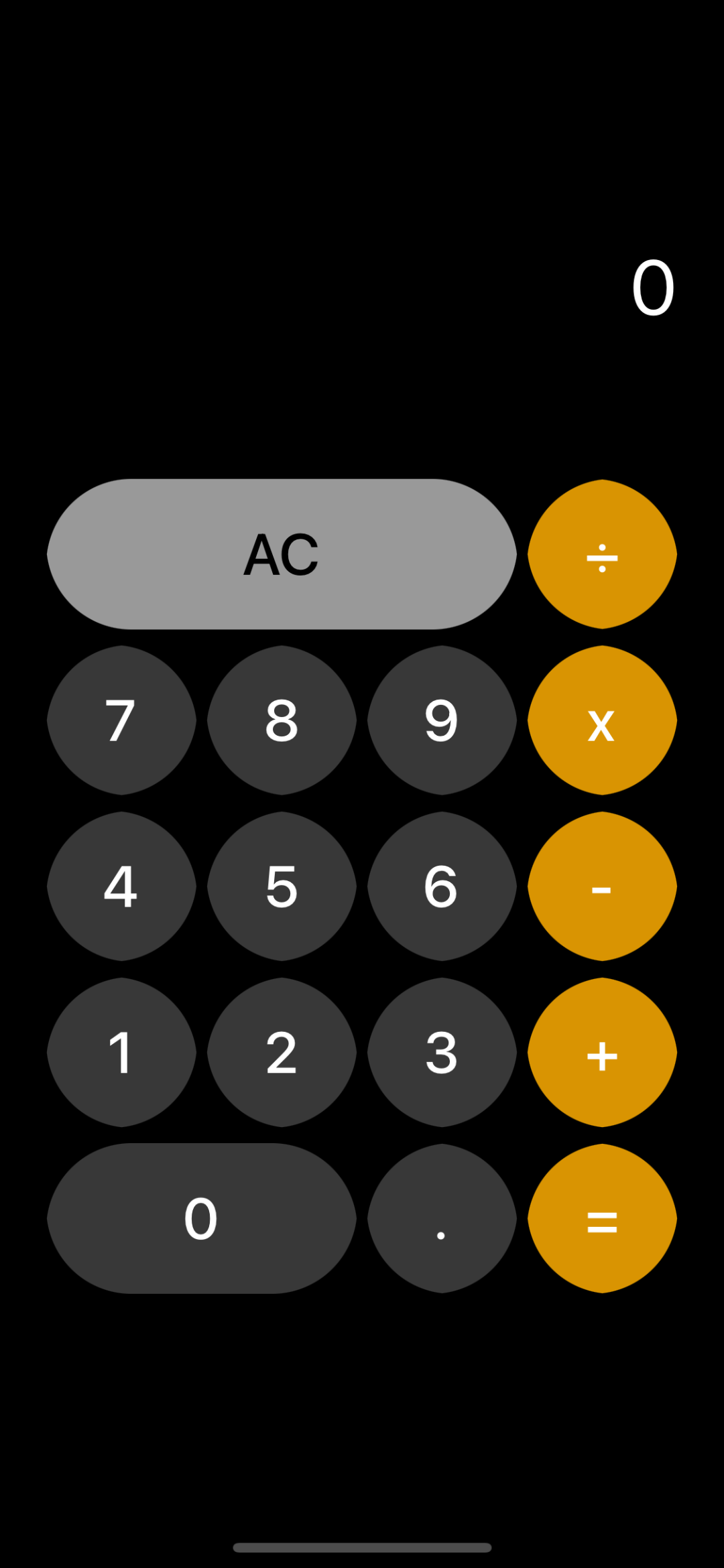The image displays a screenshot of a standard phone calculator app, currently showing the value zero. The screen is devoid of any ongoing calculations. Interestingly, the app's name is not visible, and there are no typical phone menus or status icons such as time, battery level, signal strength, and navigation buttons at the top or bottom of the screen. The calculator features a typical layout set against a black background.

The button labeled "AC," which is about three buttons in length, appears in a gray tone. Positioned to the right are the function buttons for division, multiplication, subtraction, addition, and equality, each represented by an orange circle. The numerical buttons (1 through 9), including a period, are in gray and presented as single-size circles. The zero button, distinctively, is about twice the length of the other number buttons.